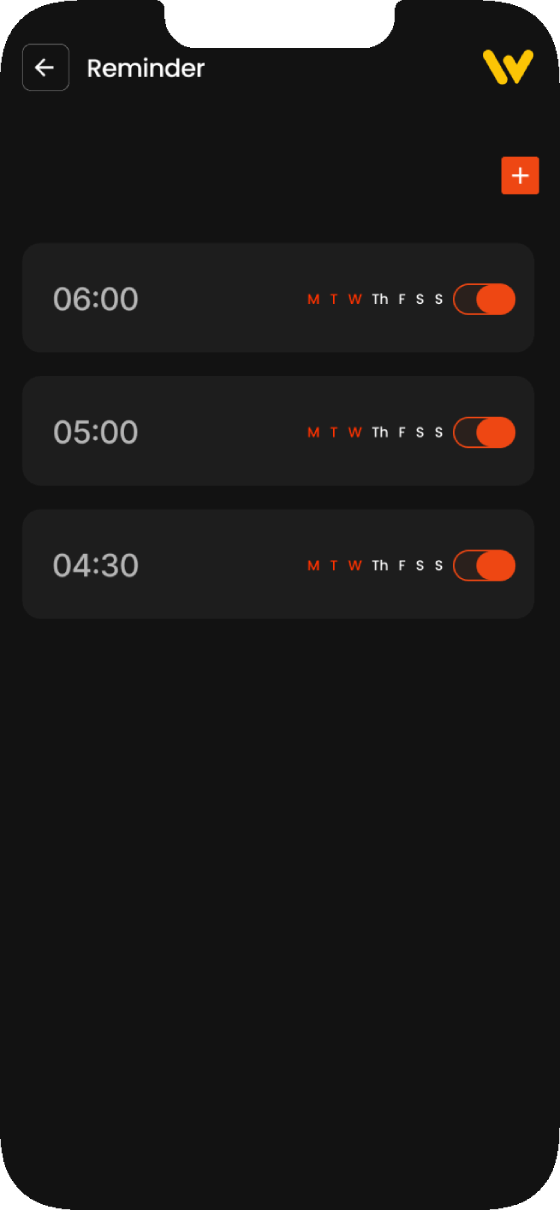The photo captures a smartphone displaying a reminder app in dark mode. At the top left corner of the screen, a white arrow pointing left is visible, followed by the text "Reminder" in white. On the top right corner, there is a yellow "W" logo. Below, a red box with a white plus sign indicates the option to add new reminders. Three reminders are listed beneath this section: one set for 6:00, another for 5:00, and the last for 4:30. Each reminder is enabled, marked with a red tick on the right side. The reminders are scheduled for Monday, Tuesday, and Wednesday, highlighted in red, while Thursday, Friday, Saturday, and Sunday are not selected, displayed in white. The app's background is black, consistent with dark mode.